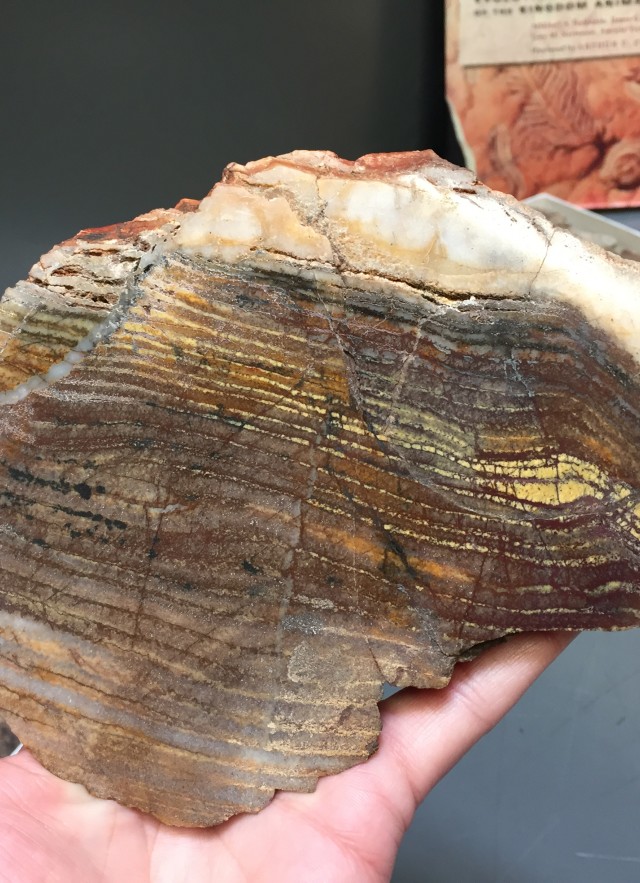This is a color photograph that possibly originated from AI creation. In the bottom left corner, part of a hand and one finger are visible, likely holding an unusual object. The background is grey, becoming darker towards the top. The object in the hand appears to be a distinctive piece of rock or possibly wood, characterized by its brown color with interspersed yellow streaks. It exhibits numerous horizontal layers, resembling the growth rings of wood, signifying an accumulation over many years. Toward the top of this object is a broken white section, adding an intriguing contrast. The overall appearance of the object, with its layered texture, brings to mind the image of a slice of iced cake in an almost surreal manner. In the upper right corner of the image, there's a sign with indecipherable black and red writing on a white background. Below this sign, a reddish object with swirling patterns can be seen, though its exact nature is unclear.